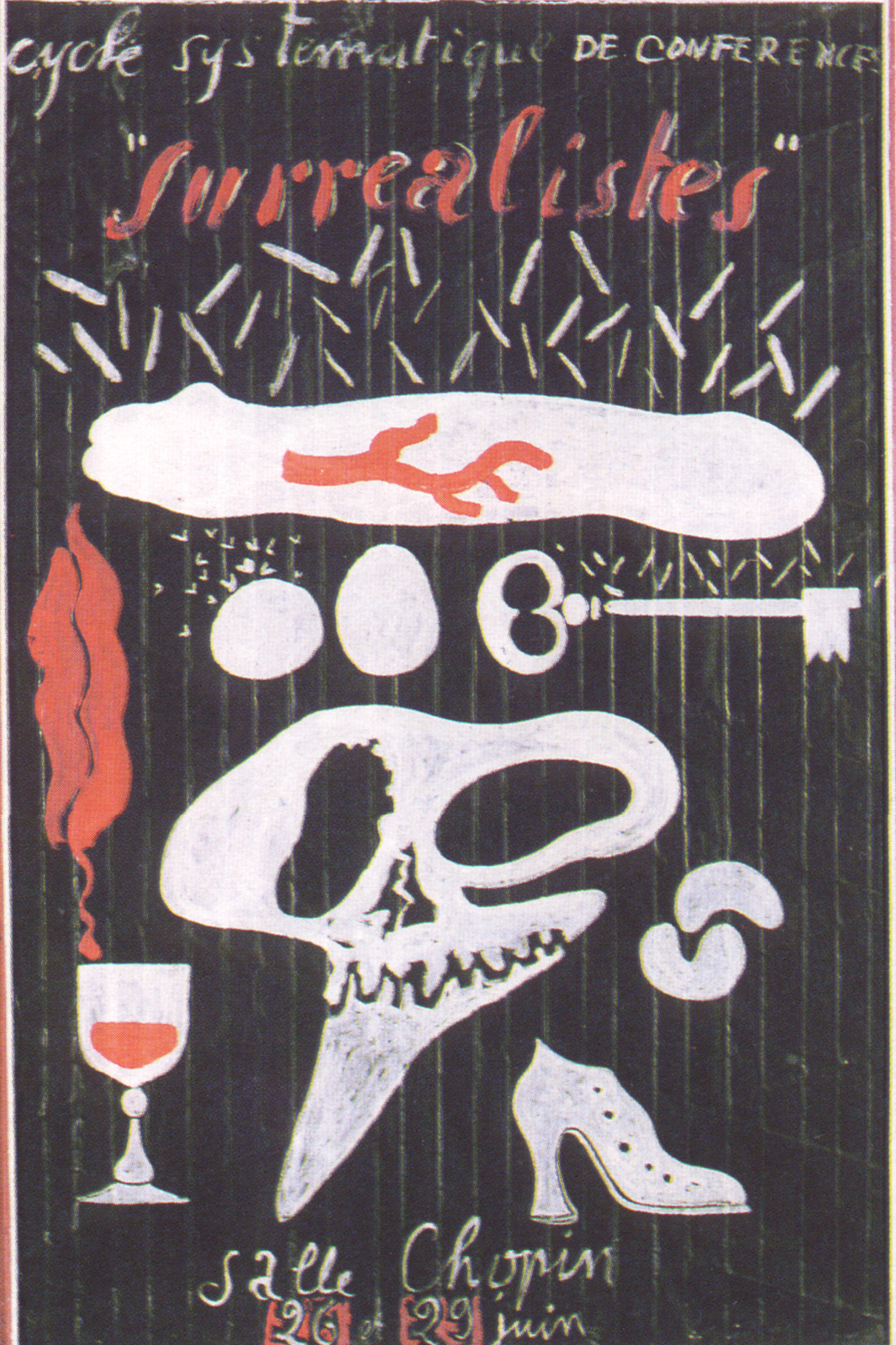In the image titled "C-Y-O-T-L-T-E," we observe a complex and surreal scene that appears to blend elements of an announcement or artistic poster. The background is primarily black, accentuated with vertical white or gray lines. At the top of the image, the title "Systematik DE Conference" is prominently displayed. Below this, the word "Surrealistist" is written in striking orange text. Beneath this text are several white lines, leading down to an irregularly shaped horizontal white section. Within this section, an orange vein-like branch or root is visible.

To the left, a white glass filled with a vivid orange drink is depicted, emitting orange flames or vapor. Centrally positioned in the image, there is a ghostly visage with two large, irregular eyes and a z-shaped mouth, introducing a spectral element. On the right side of the ghost, a high-heeled shoe is discernible.

The bottom of the image features various abstract objects: an old-fashioned key, an oddly-shaped skull, and additional elements like a bone through which a red vein courses. The word "Sal Chopiri" is inscribed at the bottom, adding to the surreal and cryptic nature of the composition. The overall effect is one of uncanny surrealism, merging disparate elements in a manner that challenges the viewer's perception.